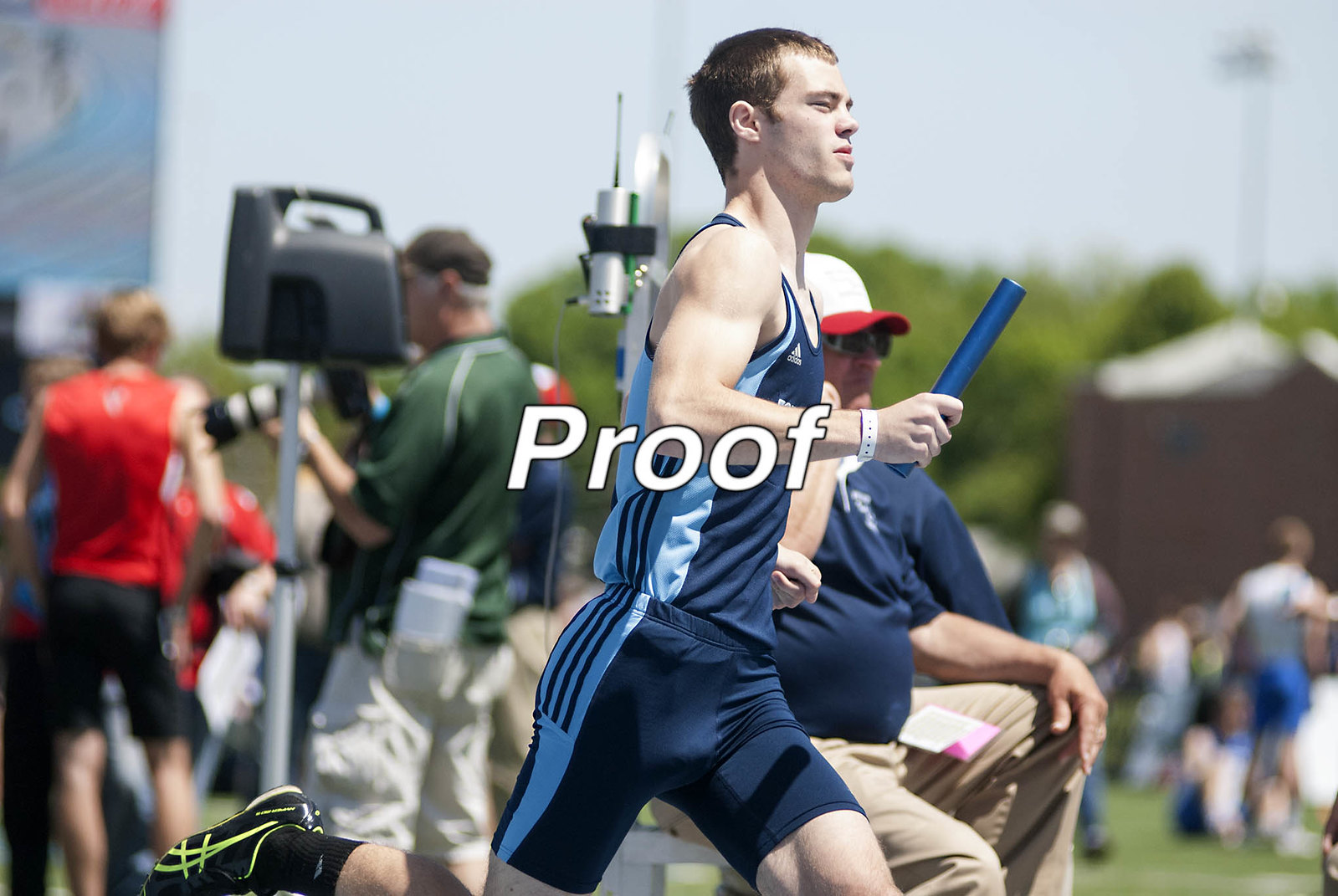The photograph captures a young Caucasian man, likely in his early 20s, running towards the right in what appears to be a track event. The primary subject is dressed in a navy blue Adidas sleeveless tank top and matching shorts, both accented with light blue panels and signature black stripes. His right leg is mid-stride, showcasing his black Asics shoes with neon yellow accents and white soles, complemented by black socks that extend above his ankles. The runner's right wrist sports a white perforated wristband, and in his hand, he grasps a cylindrical blue baton. 

He has short brown hair and is visibly well-defined in terms of physical fitness. The background features a blurred crowd, including a man in a navy shirt, khaki pants, and a ball cap sitting down, as well as other spectators or participants who are out of focus. The sky overhead is light gray, suggesting the photo was taken during the day, with some greenery and trees also present in the scene, creating a vibrant but slightly diffuse backdrop.